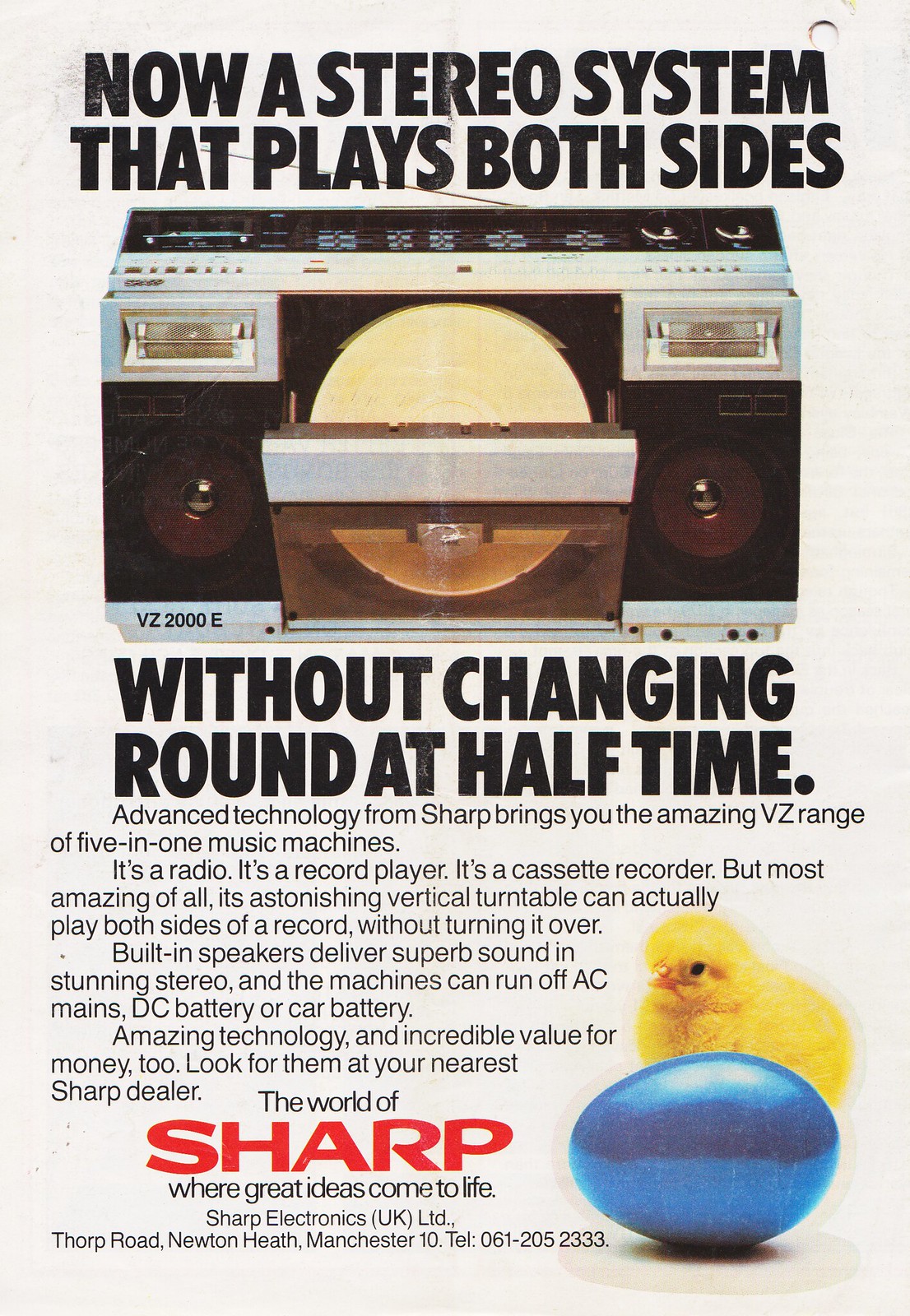The image is a poster featuring an advertisement for a stereo system. At the top, bold capital letters proclaim, "NOW A STEREO SYSTEM THAT PLAYS BOTH SIDES." Below this, there is a detailed photograph of the stereo system, which has the appearance of an old-style boom box. The front of the stereo system is brown with transparent glass or plastic, and the controls are situated on the top.

Underneath the photograph, more text reads, "Without changing round at halftime." Further down, smaller letters elaborate, "Advanced technology from Sharp brings you the amazing wizardry of 5-in-1 music machines. It's a radio, it's a record player, it's a cassette recorder, but most amazing of all, its astonishing vertical turntable can actually play both sides of a record without turning it over. Built-in speakers deliver superb sound in stunning stereo, and the machines can run off AC mains, DC battery or car battery. Amazing technology and incredible value for money too. Look for them at your nearest Sharp dealer. The world of Sharp where great ideas come to life."

Towards the bottom right corner of the image, the company name "Sharp" is prominently displayed in large red letters. Adjacent to the text, there is a blue egg with a yellow chick peeking from behind it, likely representing the logo. Further details include, "Sharp Electronics, UK Limited, Thorpe Road, Newton Health, Manchester 10, L061-205-2333."